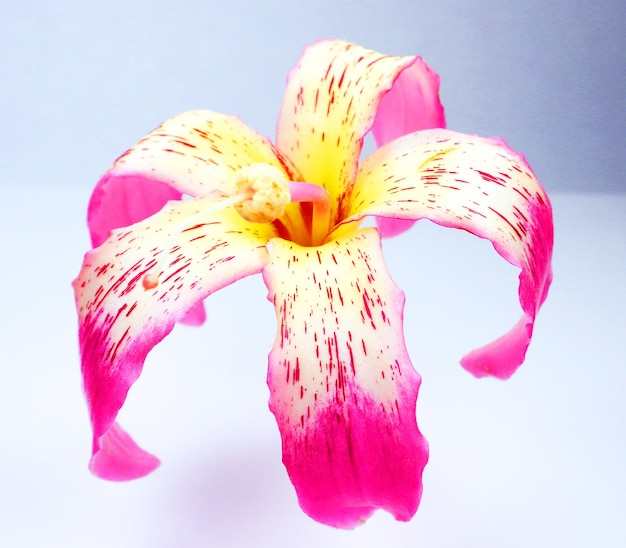This landscape-oriented image captures a close-up of a lily bloom set against a solid white background, giving a floating appearance. The flower, comprised of five long, drooping petals, displays a captivating gradient: the petal tips are a vibrant pink that flows inward into white adorned with delicate pink stripes, which gradually transitions into a beige cream before culminating in a deeper yellow at the core. The flower's stamen, positioned centrally, is a vivid yellow, adding depth and contrast to the detailed proximities of the petals. The image, likely taken indoors, shows no stem or leaves, and the overall setting is minimally disturbed except for a darker shadowed corner in the upper right, emphasizing the flower’s vivid hues and intricate patterns.